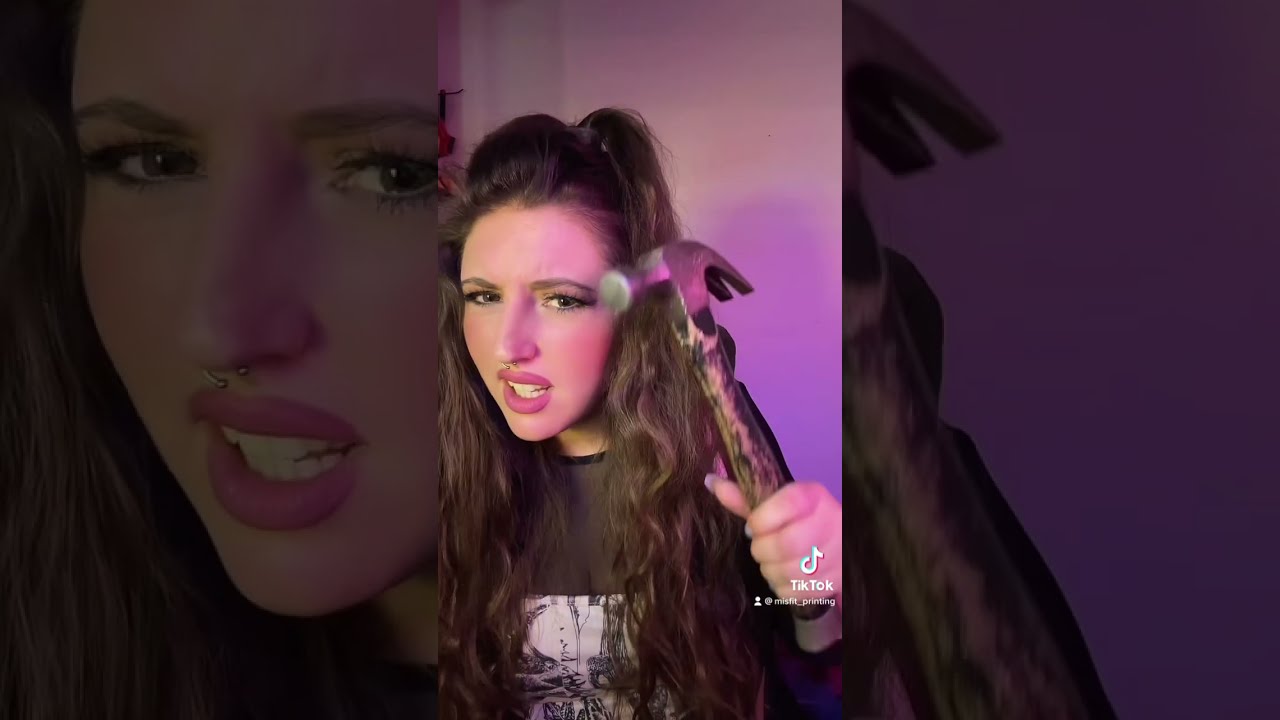In this vertical still frame from a TikTok video by the account Misfit_printing, a white girl with long brown hair pulled back in a ponytail and extending past her chest is featured in the center portion of the image. Her makeup is nicely done with pinkish lipstick, and she sports a small nose ring. The girl, illuminated with a purple or pink tint, is wearing a black shirt with a white rectangular patch bearing a black and white design on it. She has an expression that appears a bit angry or disgusted and is holding a hammer up in her left hand, seemingly poised to strike. The left and right sides of the frame zoom in on parts of the central image, with the left focusing more on her face and the right highlighting the hammer, both sections darker. The image has a Gothic or 90s vibe, with the TikTok logo and account name displayed in the bottom right corner.